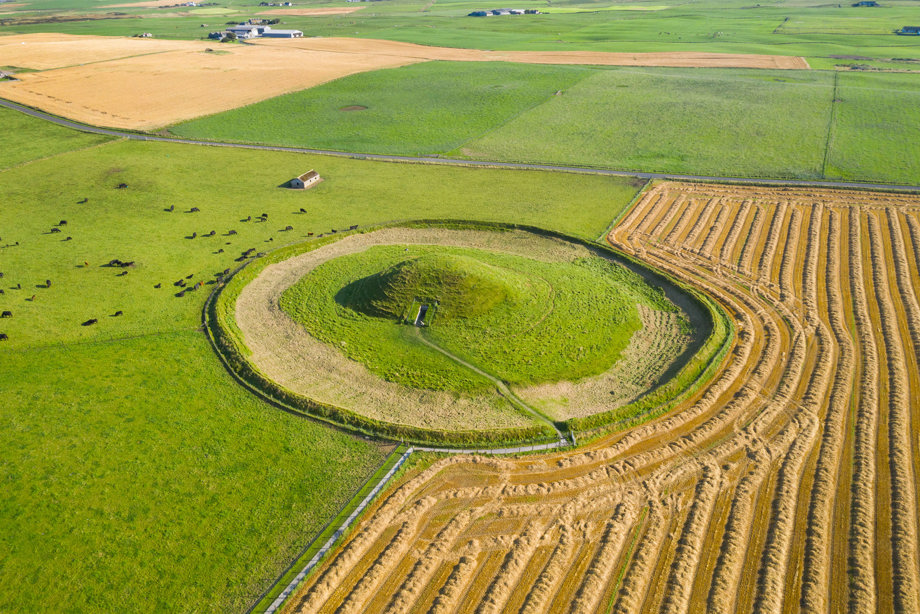This aerial image captures an expansive farmland scene, detailing both agricultural and pastoral elements. The left side of the picture showcases fields that have been meticulously plowed and partially harvested, with neat rows of cut hay straw evident. Towards the center of the image, there's a distinct round circle with an earthen mound at its center, which appears to be a water well or cellar. A trail extends from this mound, potentially indicating a drainage system. Additionally, more fields of clear green grass can be seen to the right, housing herds of cattle or sheep. A road bisects the area, separating the plowed sections from other green pastures, and a barn is visible adjacent to the fields where livestock graze. The predominant colors in the scene include varying shades of brown and green, along with specks of black and white, depicting the natural elements and agricultural use of the land. The absence of sky in the image further highlights the detailed landscape below.